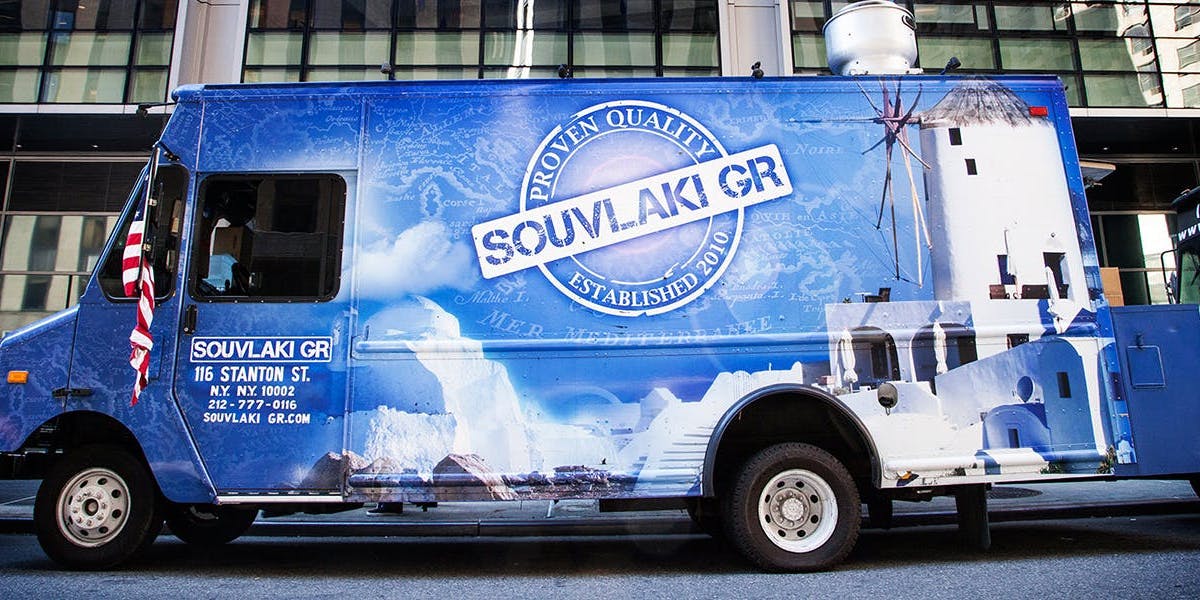This image depicts a delivery van belonging to the brand "Souvlaki GR." The van features a striking royal blue and white color scheme. Prominently displayed on its side is an image of quintessential whitewashed, white stone buildings characteristic of a scenic Greek island, set against a vividly bright blue sky. At the center of this image lies a circular emblem with the phrase "Proven Quality Established 2010" inscribed within it. Overlapping this circle is a white banner bearing the brand name "Souvlaki GR" in bold print. The van's door is equipped with a square glass window, and an American flag, partially rolled up, hangs from the front driver's side window. The vehicle is parked outside what appears to be a corporate building in an urban setting.